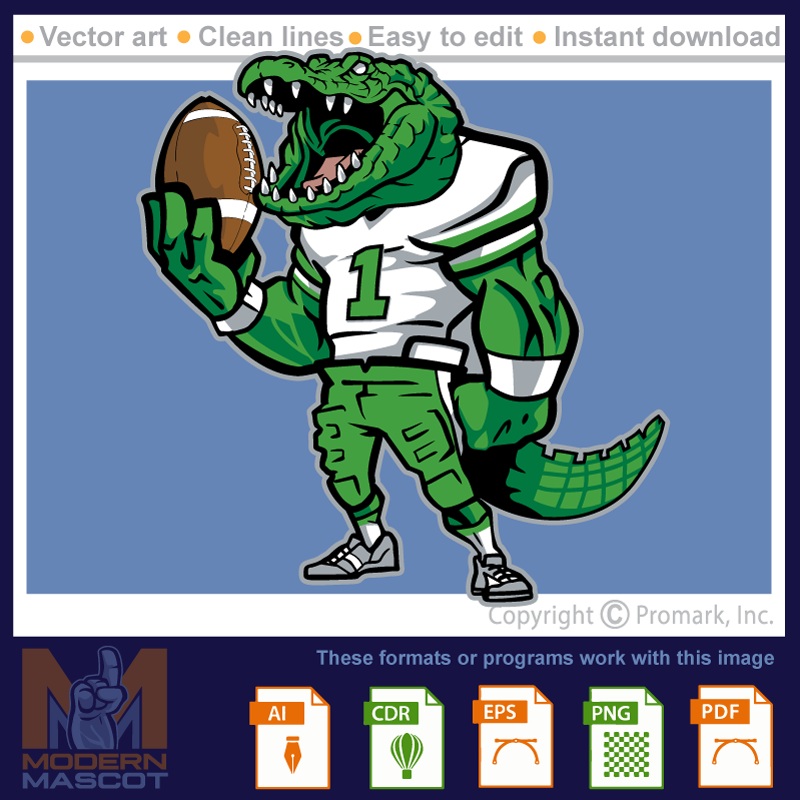The image illustrated is a detailed vector art advertisement created by Modern Mascot, showcasing a cartoon-like, computer-generated graphic of an anthropomorphic alligator football player. In the center of the image, set against a white background surrounded by a dark blue border, the alligator character is prominently featured. The alligator has a human body with a green alligator head and tail, and it is clad in a white jersey with the number one in green, white armbands, and gray shoes. The character holds a football in its right hand, poised as if about to bite it, and its left hand is balled into a fist.

Text at the top of the image, each word separated by an orange circle, reads: "Vector Art," "Clean Lines," "Easy to Edit," and "Instant Download," in a basic gray font with each first letter capitalized. In the bottom section, the available file formats are listed as AI, CDR, EPS, PNG, and PDF, indicating compatibility for instant download and edit. The bottom left corner features the Modern Mascot logo, depicting an "M" with a finger pointing up, symbolizing being number one, and the text "Modern Mascot." Additionally, below the mascot's left foot, there is a copyright mark noting "Pro-Mark Ink."